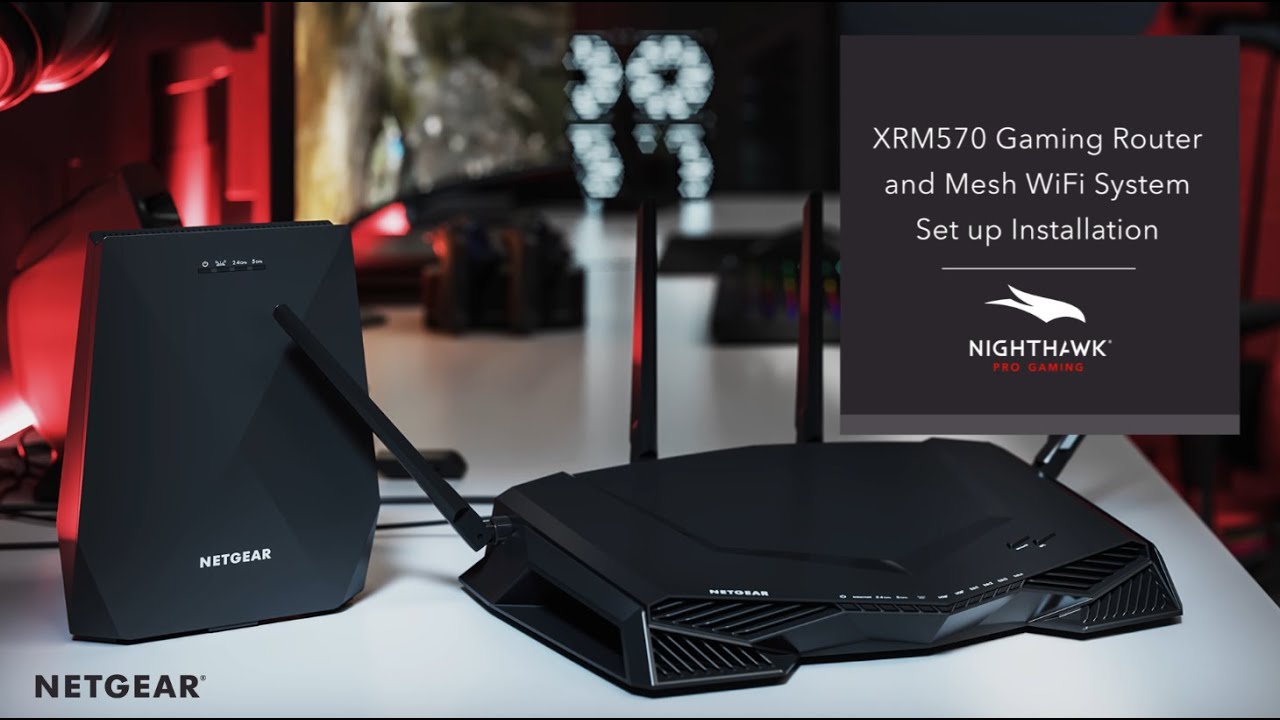The image is a high-quality product photograph intended for commercial use on online shops, catalogs, or websites. It showcases a sleek, black Netgear router and modem, designed with an edgy, gamer aesthetic, placed on a clean, light gray table. The photograph is oriented in a rectangular format, approximately six inches wide and four inches high, with thin pinstripe black horizontal lines running from the top left to the upper right corner, and from the bottom left to the bottom right corner. In the top right corner, a black rectangle with white text prominently reads "XRM570 Gaming Router and Mesh Wi-Fi System Setup Installation," followed by the Nighthawk Pro Gaming logo. The bottom right corner features black text that reads "Netgear." The background is blurred with some red and blue lights, adding a subtle but dynamic ambiance. The overall styling emphasizes the modern, high-performance nature of the Netgear gaming router and mesh Wi-Fi system.